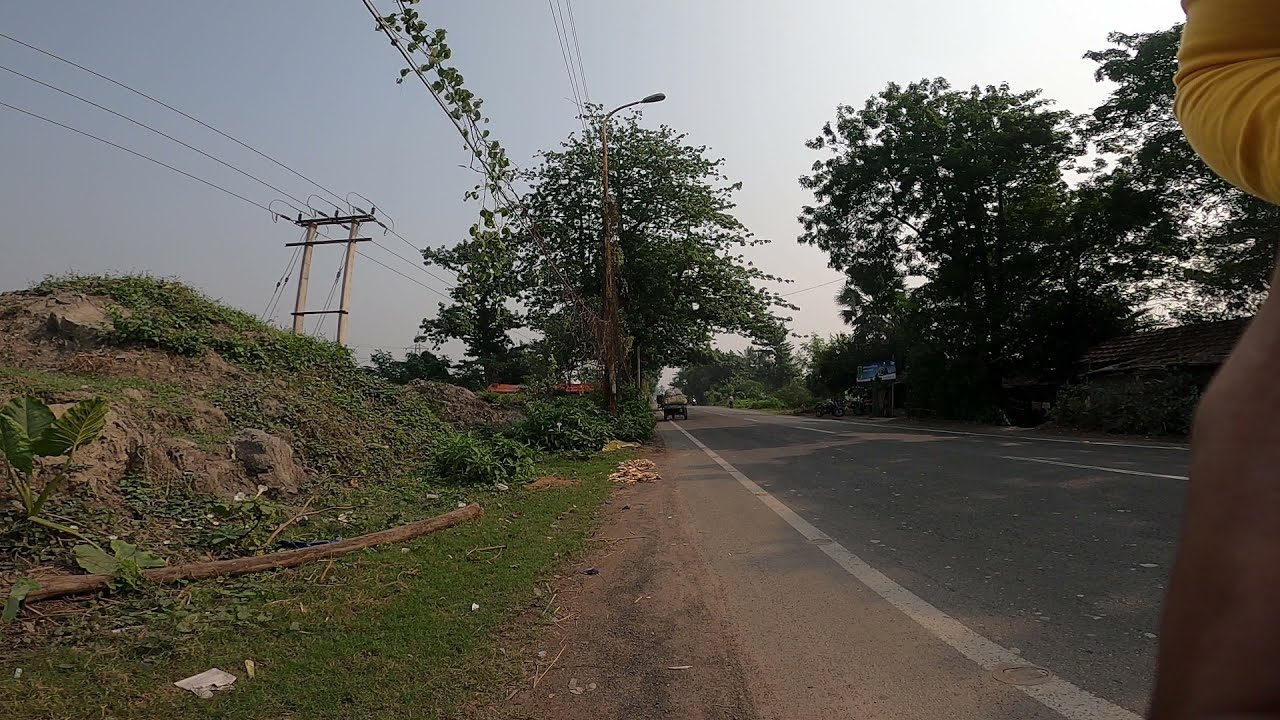The photograph is a detailed color exterior daylight view of a road captured from the side. On the right-hand side of the image, a person’s arm, clothed in a yellow long-sleeve shirt, partially appears, with an exposed knee and elbow visible. The road, a gray, two-lane asphalt highway, features a broken white stripe down the middle and solid white stripes on the edges. To the right of the highway, there are tall green trees and a low-lying building under them. Near this building, a blue and white sign partially obscured by vegetation is visible. Above the road, multiple power lines stretch across poles, some of which are overgrown with green vines. In the distance, on the left side, there are more power lines supported by a large electric tower. Further left, there is a hilly area with grass, bushes, and exposed stones. A military-type truck loaded with goods navigates down the highway, while another vehicle is parked by the side of the road. The pale blue sky envelops the entire scene.